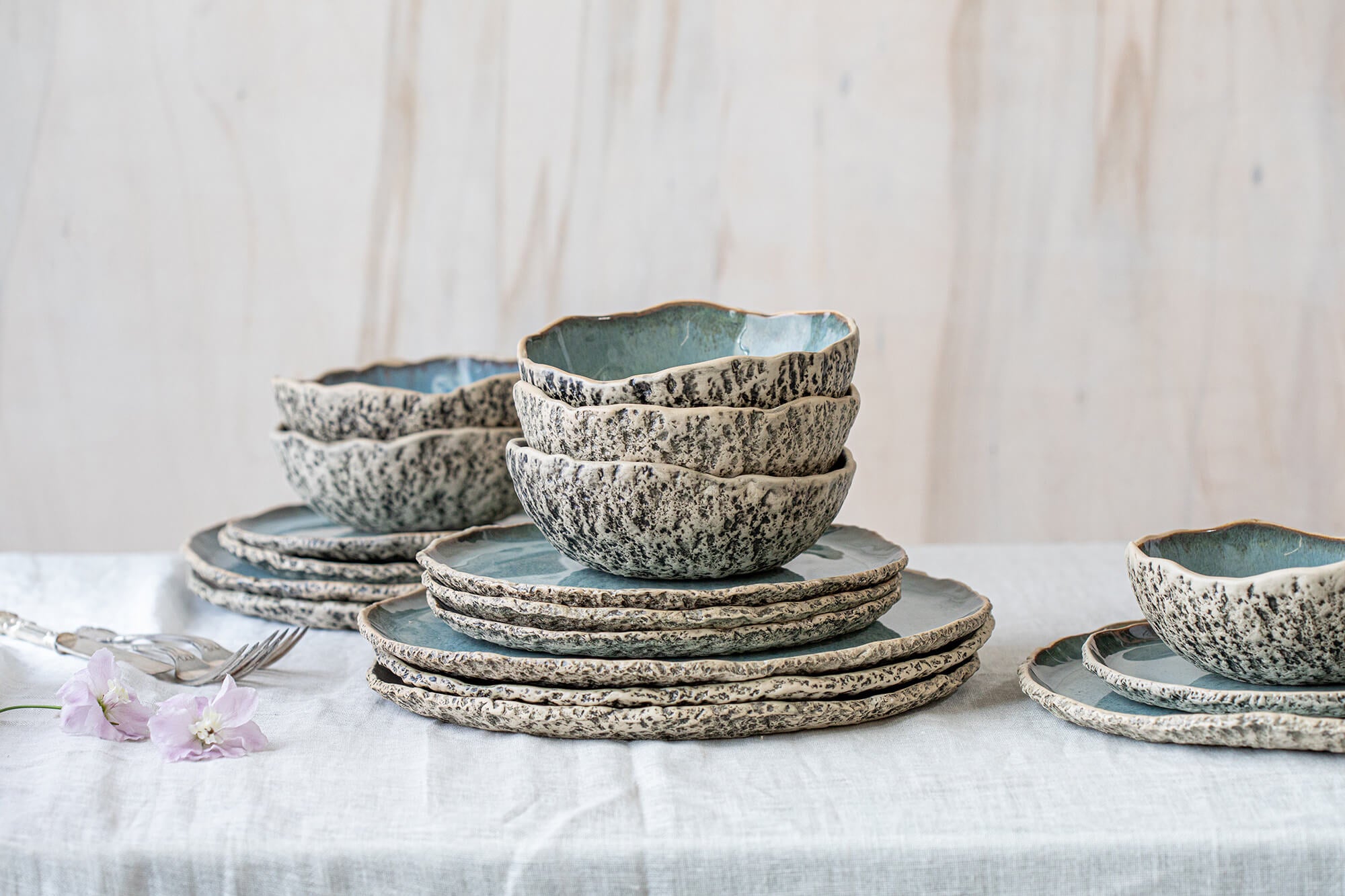The image depicts an elegantly set table covered with a white tablecloth, resembling a cheesecloth or muslin fabric. The background appears white with subtle tan streaks, creating a marble-like effect. At the center, there are multiple stacks of hand-crafted, glazed ceramic dinnerware. The dinnerware includes large and small flat plates, all sharing a rough, bony texture with scalloped edges that appear uneven, enhancing their handmade appeal. The plates are predominantly white with brown and black marbling, and their inner surfaces showcase a striking greenish-blue hue. 

Specifically, there are three stacks of dinner plates, each consisting of a trio of large plates topped with smaller plates and bowls. Two similar stacks are positioned on the left side of the image, and a single set is placed to the right. The bowls, matching the plates in design, sit gracefully atop each stack. Additionally, there are stainless steel forks and knives grouped together, accompanied by light purple flowers, which add a touch of softness and color to the otherwise neutral-toned setting. This visual arrangement speaks to a harmonious blend of rustic elegance and artistic craftsmanship.